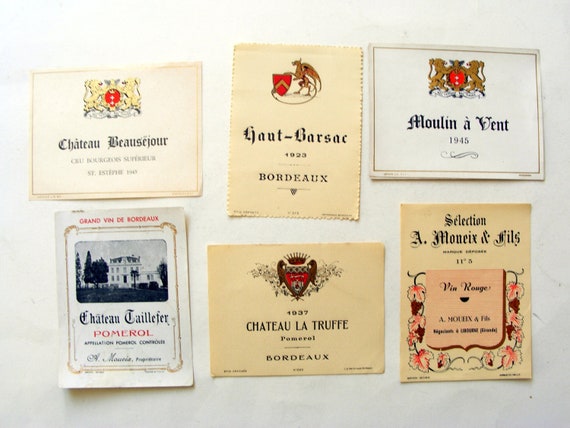The image showcases six beige or white wine bottle labels, all written in French and appearing to be from various chateaux, each with its distinctive emblem. The labels are meticulously arranged, with five of them longer than they are tall and one that is taller than it is wide. Each wine label features a unique crest or emblem at the top, followed by the chateau name prominently displayed in the center, with additional details including the year of vintage below.

Starting from the top left, the first label displays two golden lions facing each other with a red shield between them, and mentions Chateau Beau Sejour. Next to it, the second label stands taller and features a dragon-like creature holding a shield, indicating a Bordeaux wine from 1923 by Chateau Haute Barsaque. The third label, similar to the first, shows the twin lions crest and mentions Chateau Califre, with the notable vintage year of 1945.

In the bottom row, starting from the right, the fourth label is tall and narrow with dark text at the top, showcasing a pink centerpiece framed by vines and leaves. To its left, the fifth label is shorter and says Chateau La Truffe, bearing the year 1937 and a badge at the top. Finally, the sixth label is long and narrow, adorned with a black and white depiction of a building at the top and surrounded by a bordered frame.

These six wine labels, seemingly from some rare and prestigious French wines, combine the elegance of their respective emblems with clear, bold text, illustrating a rich history of vintages.